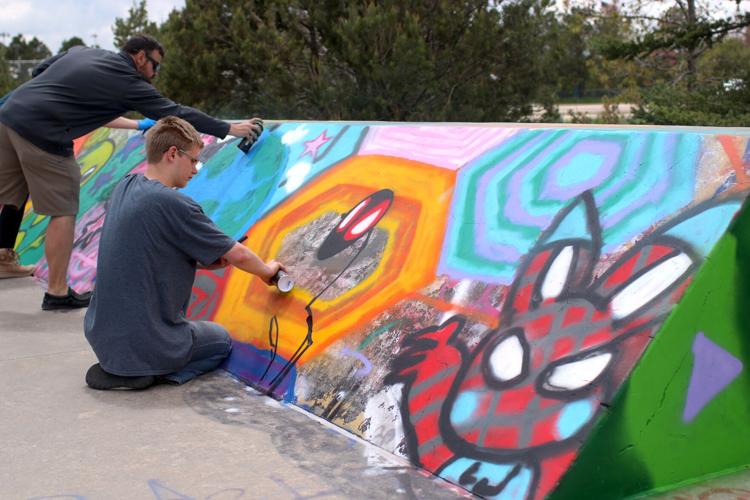In this image, two young men are engaged in spray painting an outdoor triangular structure, possibly a part of a skate park or a large angled wall. They are positioned on the left-hand side of the photo. The man standing in a gray shirt, tan shorts, mismatched shoes (one black, one tan), and sunglasses is bent over, spraying a blue section near the top. He has brown hair. Next to him, a kneeling man with dirty blonde hair styled in an undercut, glasses, a dark gray t-shirt, and blue jeans, is painting a yellow section. Their surroundings include daytime skies with blue clouds and trees in the background. The artwork they are creating features a black alien-like face with large, white eyes and red-green tones, alongside a cartoonish creature resembling a rabbit, also with exaggerated white eyes. The mural incorporates several geometric shapes in pastel hues, such as hexagons in blue, pink, and yellow, as well as shapes in orange, aqua, and purple. The overall scene captures the vibrant activity and creativity of street art in a dynamic outdoor setting.